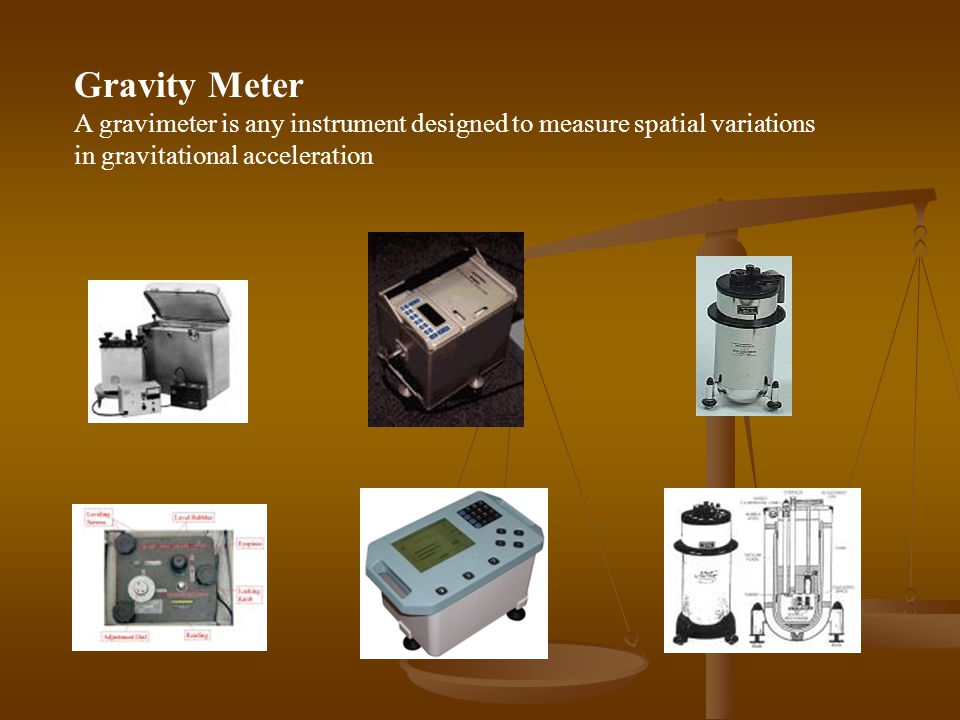The image appears to resemble a PowerPoint presentation or educational textbook page. The background features a gradient that transitions from golden yellow to lighter brown, culminating in a darker brown at the top and bottom. A blurry, 3D-rendered justice scale, akin to those held by Lady Justice, is in the background.

Prominently displayed at the top in white text is the title "Gravity Meter." Below that is an explanation: "A gravity meter, also known as a gravimeter, is any instrument designed to measure spatial variations in gravitational acceleration." Positioned above these words are six images depicting various types of gravity meters. 

The gravity meters shown exhibit diverse designs: the first two are squarish, the third is more rounded, followed by another round one which appears to be a drawing showcasing its internal structure. The final two revert to squarish designs, each differing slightly in appearance. The images feature either a white or black background, presenting a visually varied layout.